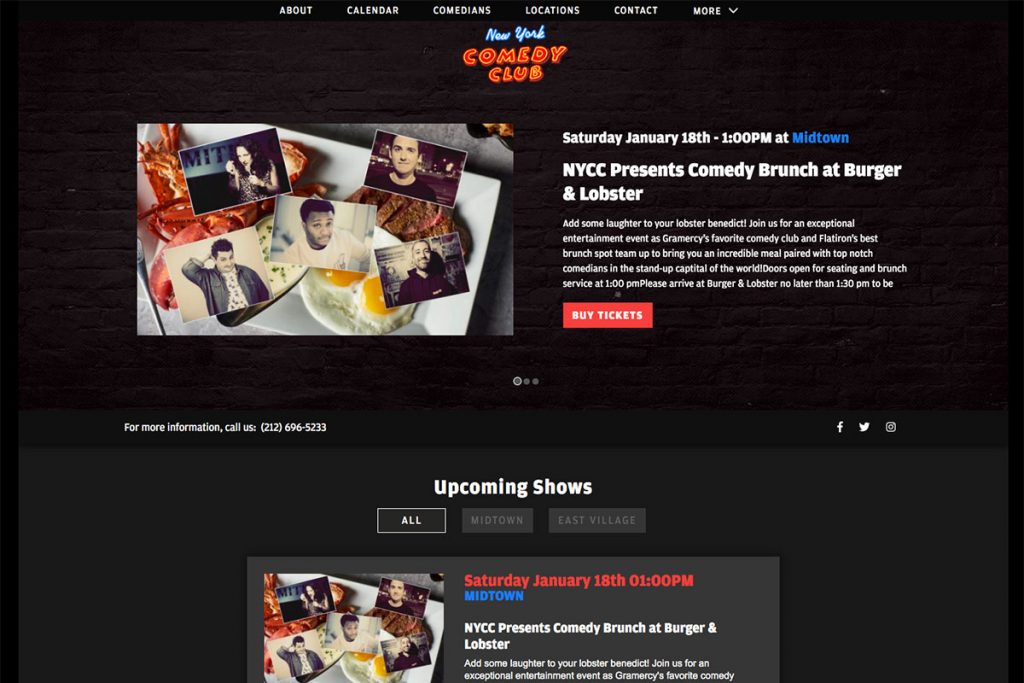This is a detailed screenshot of the New York Comedy Club's website. The logo prominently features "New York" in blue and "Comedy Club" in red, designed to mimic vibrant neon lights commonly seen in store signs. 

At the top of the page, a navigation menu is displayed with options for 'About,' 'Calendar,' 'Comedians,' 'Locations,' 'Contact,' and a 'More' dropdown menu, all written in white text and acting as clickable buttons.

The center of the screen showcases a promotional image with physical photographs of various comedians placed artfully on a plate of lobster and eggs. The text alongside this image announces, "Saturday, January 18th, 1 p.m., Midtown. NYCC presents Comedy Brunch at Burger and Lobster." 

Below the image, a call-to-action reads: "For more information, call us," followed by the phone number 212-696-5233. Social media icons for Facebook, Twitter, and Instagram are positioned to the right of this information.

Further down, a section titled "Upcoming Shows" allows users to filter events by 'All,' 'Midtown,' or 'East Village.' It is set to 'All' by default and lists the same Comedy Brunch event with the recurring image.